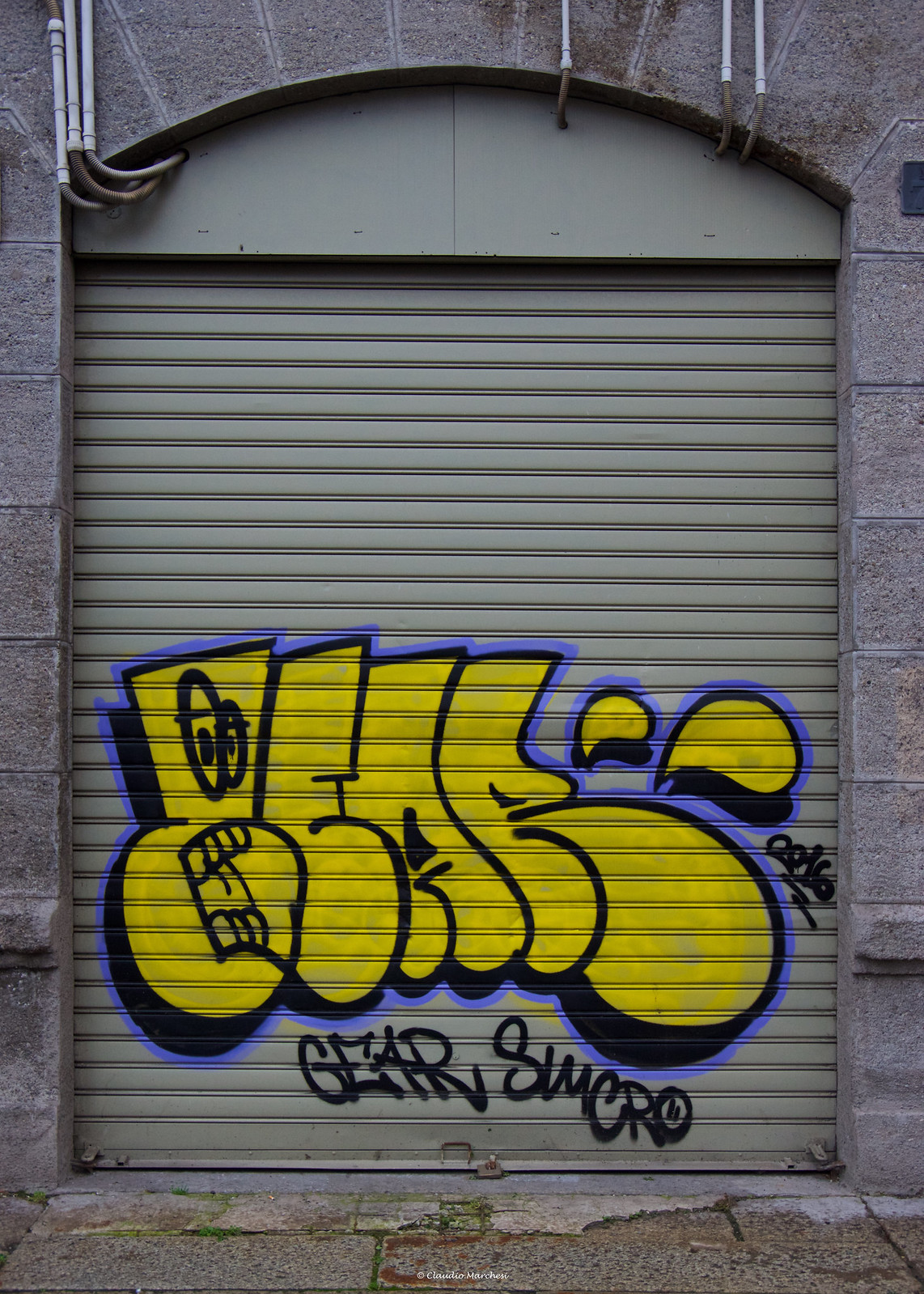The photograph shows an outdoor scene featuring a large, closed, grey metal rolling door, possibly part of a garage or storage container. The door is set within a grey stone or cinder block building, which has an arched top structure composed of stone bricks and some pipes extending from the archway. The ground at the base of the door is also made of stone.

Prominently displayed on the door is vibrant graffiti, characterized by bold yellow bubble letters outlined in black and further accentuated by a purple outline. The text spells out "Gear" with a creative twist—the 'G' is personified, featuring cartoon-like eyes, a mouth with teeth and a tongue, and two droplet icons emerging from its right side. Below this, in black text, it reads "gear Simcoe," with the 'O' depicted as a face with two dashes for eyes.